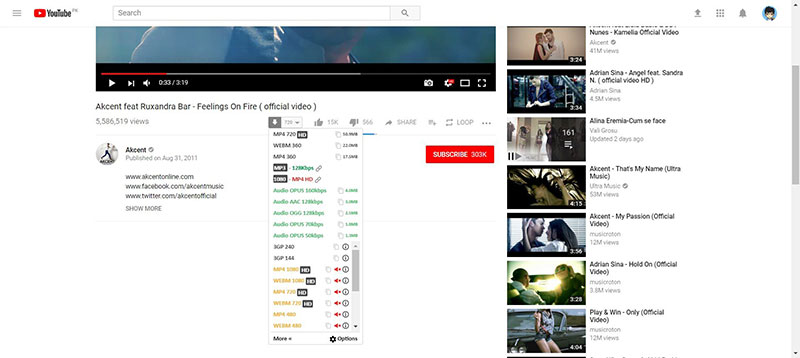This detailed image taken from YouTube displays the platform’s interface. Dominating the screenshot is a large red square featuring the iconic white play button, symbolizing the brand’s identity. At the top of the interface, there's a search bar poised to help users find content. Below this, a video is currently playing, evidenced by the partially advanced red progress bar indicating the viewer has already watched a segment of the video. 

The video’s title, "Alcent featuring Responder Dra Bar - Feelings on Free (Official Video)," suggests it’s a music video by the artist Alcent, in collaboration with Responder Dra Bar. The title implies it's an official release, adding authenticity and perhaps professionalism to the content.

On the left side of the screen, there’s a vertical dropdown bar with various menu options highlighted in green, gold, and black, providing navigational aid throughout the site. In the center-right of the screen, there's a small red bar or button that appears clickable, likely for accessing additional options or settings.

The right side is populated with a series of thumbnails showcasing "Official Trailers" and "Official Videos." Each thumbnail includes a preview image, a brief video description, and is clickable, allowing viewers to explore further content based on their interest. This layout exemplifies YouTube's organized and user-friendly interface, designed to keep viewers engaged and provide easy access to a myriad of videos.